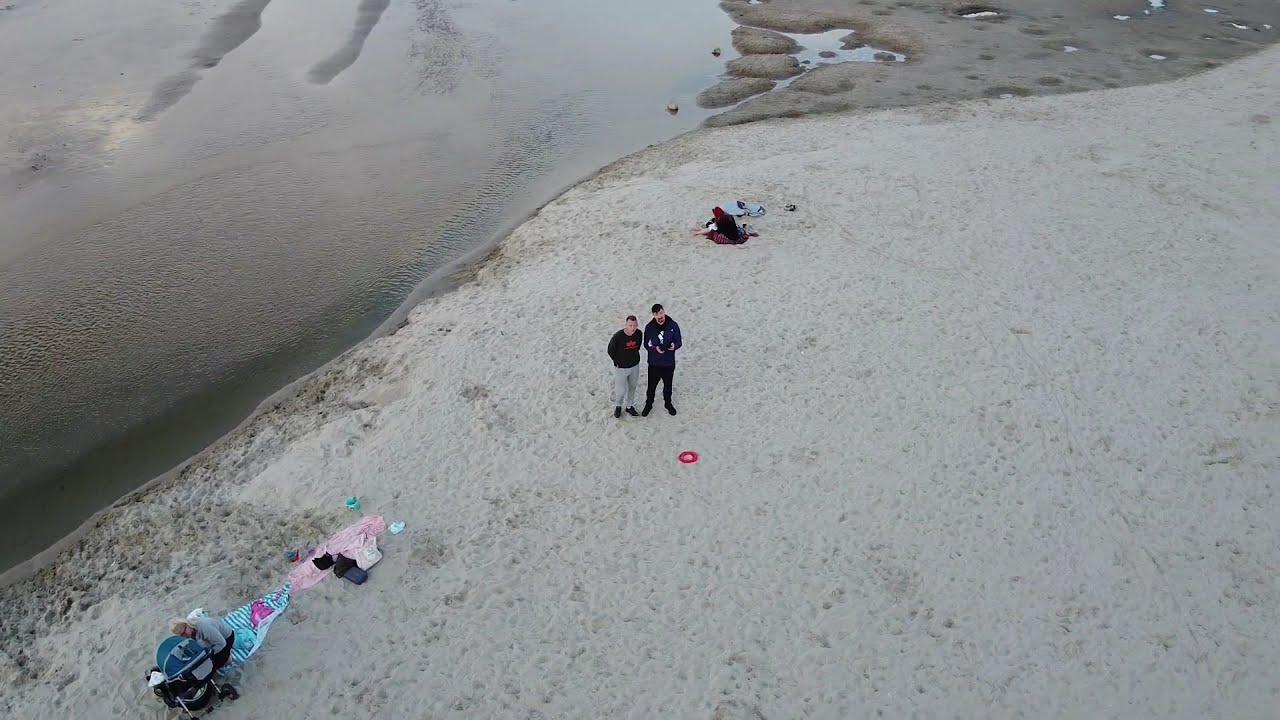The color photograph captures a bright, sunny day at what appears to be a lakeside or riverbank with a thin shoreline and some visible sandbars in the water at the upper left corner. Centrally positioned are two men standing on the sandy ground marked by a red circular indicator. The man on the right is dressed in black pants, black shoes, and a black long-sleeve shirt, and is holding a controller, likely operating a drone hovering above their heads. The man on the left sports light-colored pants, black shoes, and a black shirt, also gazing upwards. Nearby, in the lower left corner, a person is bent over a stroller positioned on a green striped towel and a pink blanket, suggesting a leisurely outing. The ground is a mix of beige and brown sand, indicating a typical beach environment with no text or numerical markings. The overall ambiance is well-lit by natural sunlight, enhancing the clarity and colors in the image.